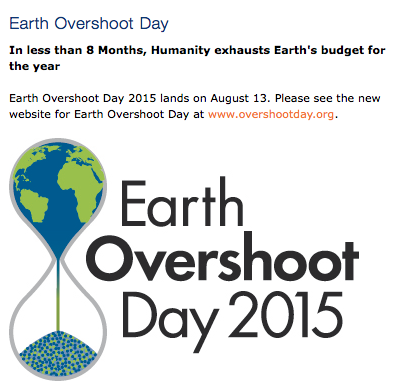This is an image of an intricately designed minute timer, reminiscent of an hourglass or egg timer, set against a stark white background. The upper section of the timer features a vibrant depiction of the Earth in blue and green hues, symbolizing our planet's natural colors. As the sand flows through to the smaller portion below, the particles maintain the blue and green colors, visually suggesting the depletion of Earth's resources. 

The image prominently displays a message in blue text reading "Earth Overshoot Day." Below, in bold black text, it states, "In less than eight months, humanity exhausts Earth's budget for the year." Further down, it is indicated that "Earth Overshoot Day 2015 lands on August 13th," highlighted in large, bold letters, underscoring the urgency of the situation.

Additionally, there is a call-to-action directing viewers to "please see the new website for Earth Overshoot Day at www.overshootday.org," with the URL marked in orange for emphasis.

The overall design of the sand timer is uniquely eye-catching, featuring a teardrop shape merging into an upside-down teardrop where the image of the Earth is positioned. The meticulous detailing of the falling sand particles enhances the logo’s visual appeal, symbolizing the gradual but relentless depletion of the Earth's resources.